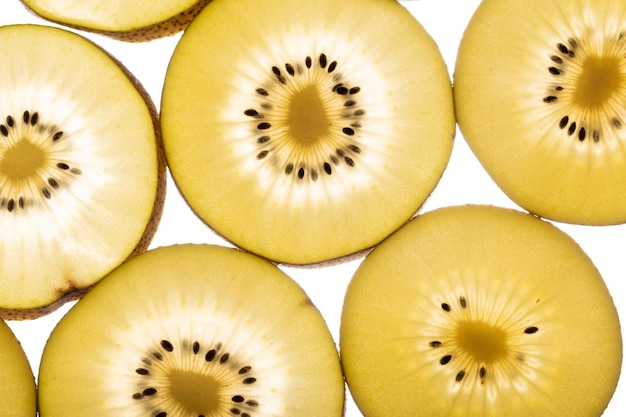This photo is a detailed, indoor, close-up shot of sliced fruit, resembling a kiwi but with distinct yellow flesh. The image, dominated by five partially visible circular slices, is set against a stark white background with no additional elements. Each slice features a dark central area, radiating with a coral-like pattern and surrounded by clusters of small black seeds varying in density. Encircling this is a white ring, beyond which the flesh transitions to a yellowish green. Some slices show hints of the outer kiwi skin. The slices are closely arranged, partially cut off at the frame's edges, and hinting at additional slices. The overall composition captures the textual and color contrasts of the fruit in intricate detail.